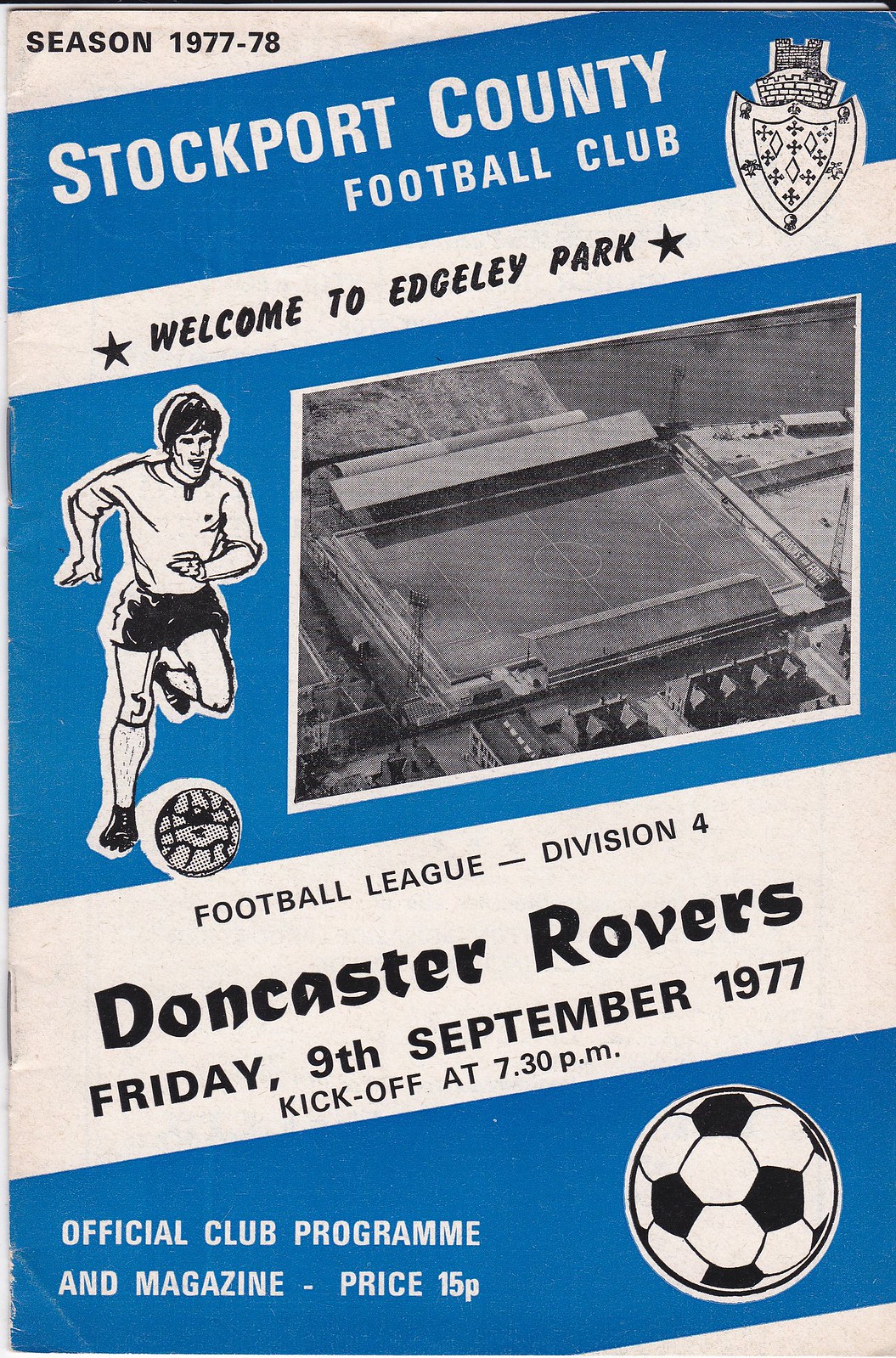The image depicts the front cover of a sports program for the Stockport County Football Club. The cover is predominantly white with several blue stripes that run diagonally across it. At the very top, in black text, it reads "Season 1977-78". Below, on the first blue stripe, is the club's name, "Stockport County Football Club", alongside a shield emblem adorned with crosses and diamonds. Beneath this, on a white stripe, the text "Welcome to Edgeley Park" is printed in black. Following this, another diagonal white banner contains a photograph of the stadium or playing field, juxtaposed with an illustration of a man kicking a soccer ball on the left. Further down, another white stripe provides details about an upcoming match with the text, "Football League Division 4, Doncaster Rovers, Friday 9th September 1977, kickoff at 7:30 p.m." Below this match information, the final blue stripe declares, "Official Club Program and Magazine, Price 15p", accompanied by an illustration of a soccer ball. The entire design suggests it is the cover of a program typically provided at soccer matches. The colors used are primarily white and blue, with black text, creating a straightforward and clean layout.